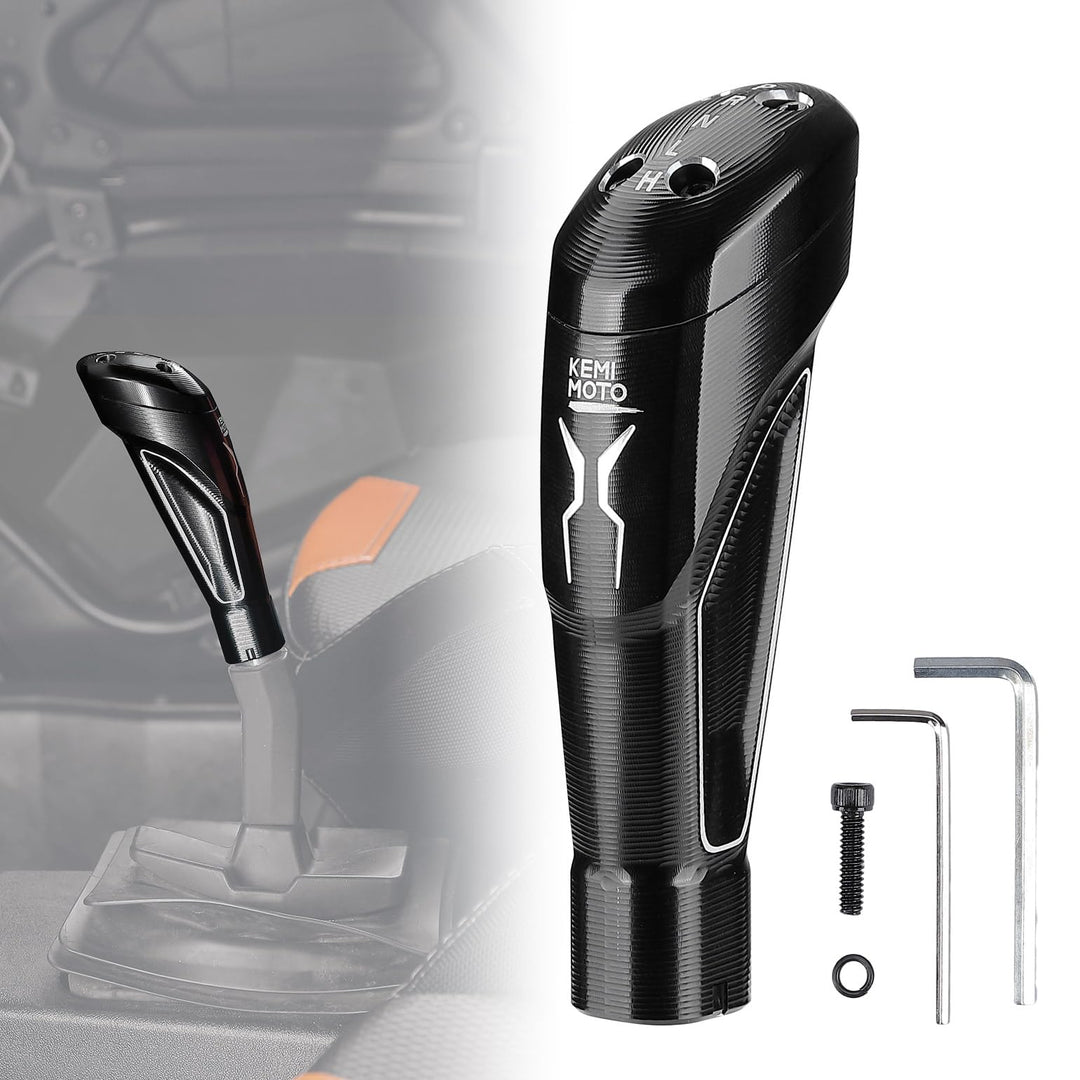The image portrays a detailed setup of a car gear shift knob and its components. At the center is a sleek, shiny black shift knob that prominently displays "Kemimoto" in white letters on its front. The top of the knob is marked with designations like high, low, and neutral. To the right of the knob are two small metal screwdrivers with plastic handles, a bolt, and a washer. These parts seem to be essential for installing or adjusting the shift knob. The left side of the image illustrates the shift knob mounted on a gear stick within a vehicle's console, alongside a partially visible orange arrow sticker that likely provides installation instructions. The shift knob appears ergonomic, intended to enhance the shifting experience in the car. Surrounding the mounted gear shift are various metal components and part of the car's interior, depicting the entire setup in a practical vehicular context.